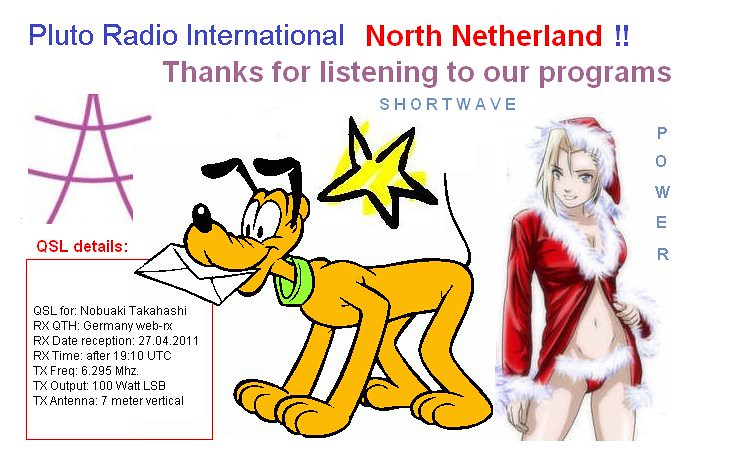Pluto Radio International North Netherlands!!

This horizontal rectangular image has a white background and is topped with the title "Pluto Radio International North Netherlands!!", where "Pluto Radio International" is in blue and "North Netherlands" is in red. Below the title, in purple text, it reads, "Thanks for listening to our programs," followed by the word "Shortwave" in blue. 

The central focus of the image is Disney's cartoon dog, Pluto. He is an orange-yellow color with black ears, a black nose, and large eyes, smiling to the left while holding a white envelope in his mouth. Pluto wears a green collar, and above him is a hand-drawn, scribbly black-outlined star filled with yellow. 

To the right of Pluto is an image of an anime-styled woman dressed in a scantily clad Santa costume consisting of a red jacket with white fur trim, a Santa hat, and revealing her belly and upper thighs. She smiles with blue eyes and blonde hair cascading over the right side of her face. Vertically aligned to the right of her is the word "POWER" in blue letters. 

In the lower left-hand corner, there is a small red-outlined box with the header "QSL details" in red. The black left-aligned text inside this box provides specific reception details: "QSL for Nobuaki Takahashi RX QTH Germany web-RX," followed by dates and technical information, including "RX date reception 27.04.2011", "RX time after 19:10 UTC", "TX Freq 6.295 megahertz", "TX output 100 watt LSB", and "TX antenna 7 meter vertical".